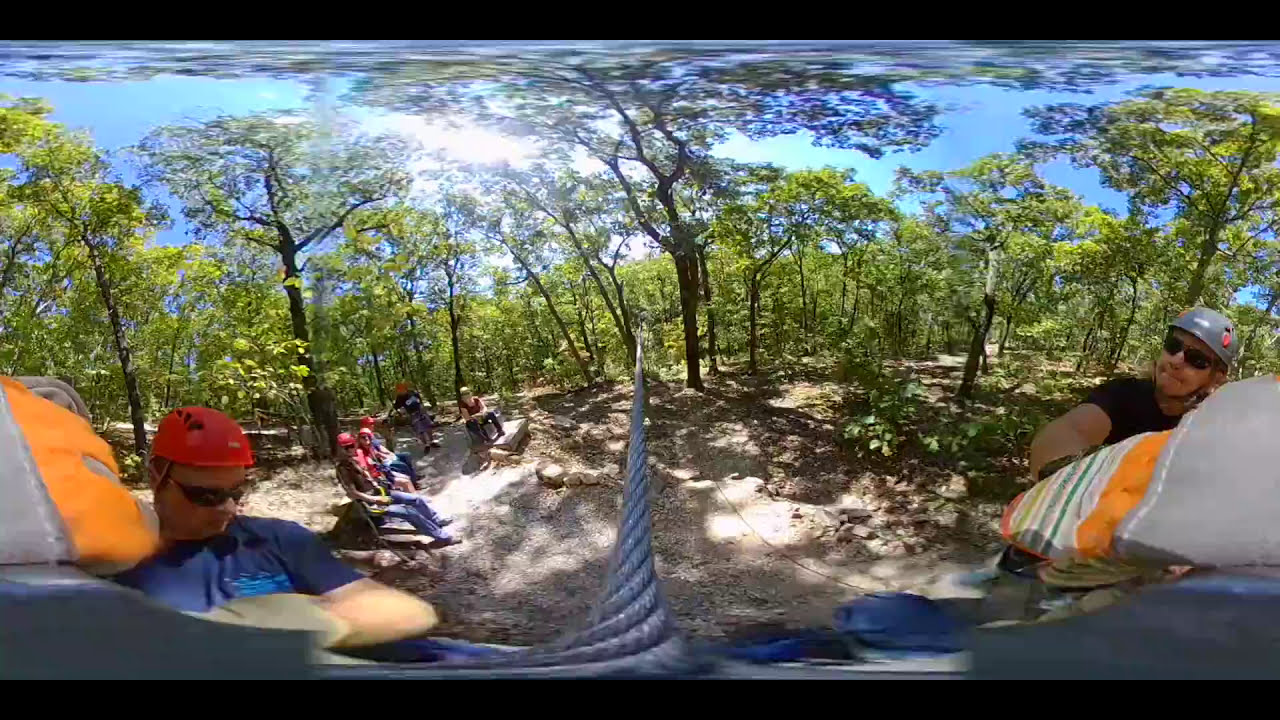The image captures a panoramic view of an outdoor zip line course set amidst a lush, tree-lined background where the green leaves and brown trunks create a natural canopy. A sturdy, steel woven cable runs centrally, likely serving as the zip line, extending from the foreground into the distant trees. 

In the middle ground, several individuals are seated on chairs directly on the dirt-covered ground, which is interspersed with gravel, rocks, and sparse patches of grass and bushes—indicating a well-trodden area. The sun casts a glow from behind the trees, adding a warm ambience to the scene.

Two individuals are prominently positioned in the image. On the left, a person is seen from the torso up, sporting a medium blue t-shirt, black sunglasses, and a light red helmet. They are facing right. To the right, another individual appears in a black t-shirt and gray helmet, with their head turned toward approximately the seven o’clock position. Both figures are central to the composition and contribute to the activity-focused narrative of the photograph. The overall setting suggests an engaging and adventurous environment perfect for zip lining.